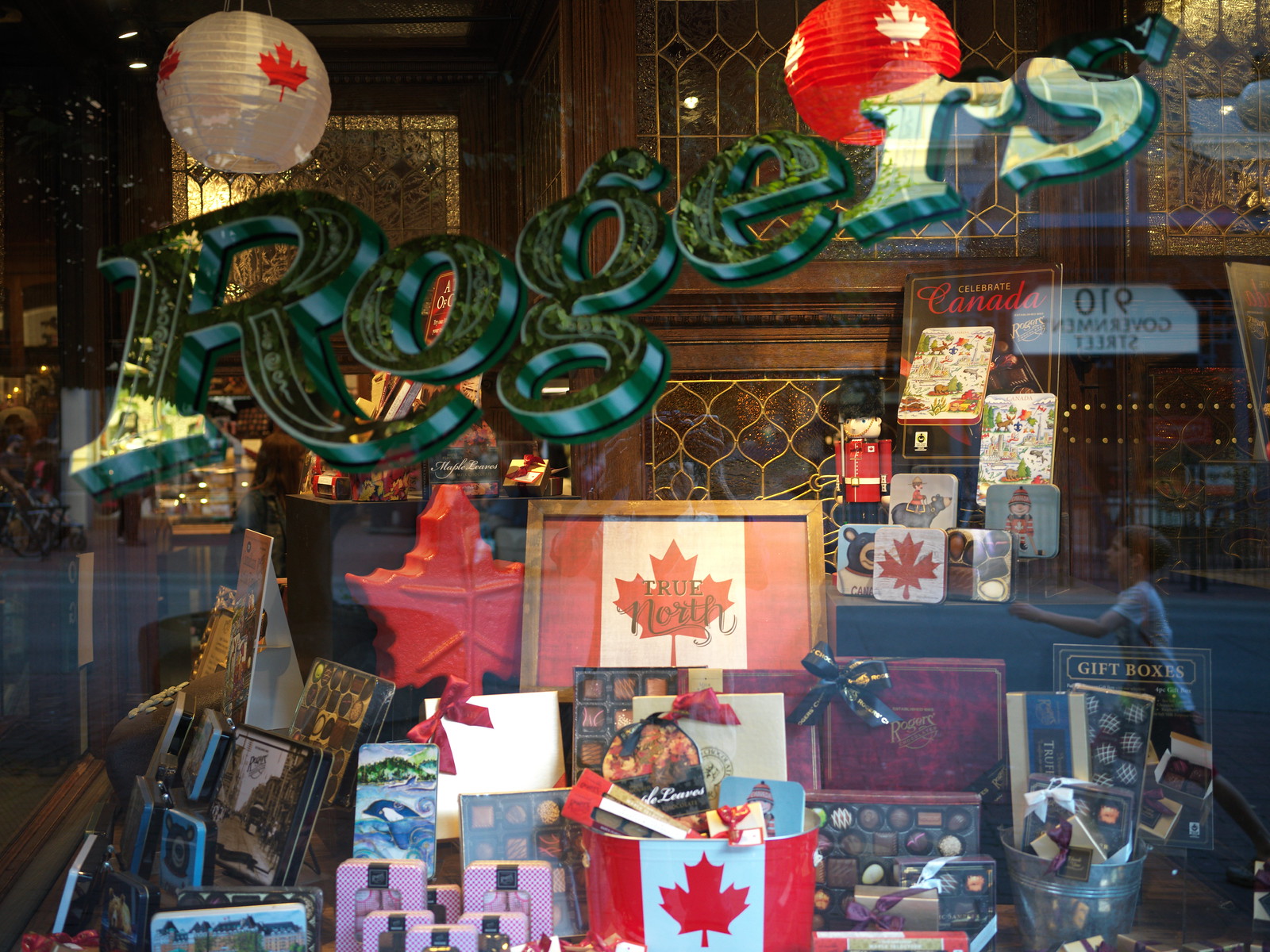This detailed photograph features the glass window of a Rogers shop, adorned with the word "Rogers" in an ornate font with green and gold letters accented by delicate decorations. The window showcases an array of items, prominently highlighting Canadian-themed decor. Visible inside are light fixtures resembling paper lanterns—one white ball adorned with red maple leaves and one red ball with white maple leaves. The display includes a tin shaped like a red maple leaf, a framed image with red and white stripes featuring a red maple leaf and the words "True North," gift items like photo frames and decorative objects, greeting cards, candies in various designs and colors, and a toy soldier. In the background, ornate stained glass windows with luxurious gold leadwork and intricate woodwork add to the visual richness. Additionally, the window's reflection offers a glimpse of the road outside, where a boy in a white shirt is seen walking.